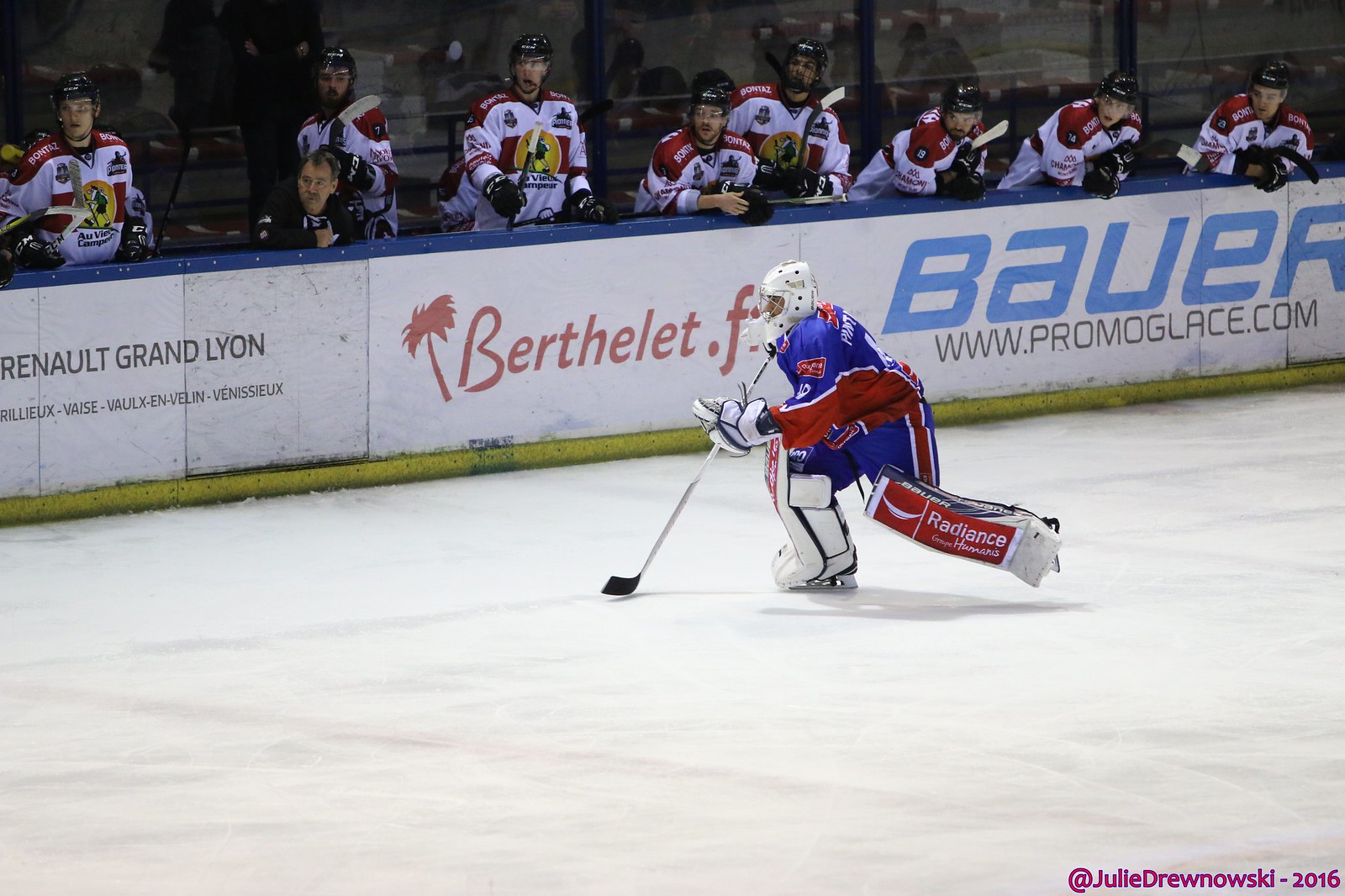The image captures a vibrant indoor setting at a hockey rink, focusing on a prominent player on the ice. The player is attired in a royal blue and red uniform, complete with leg pads, gloves, and a white helmet. He is depicted skating with his hockey stick held in front of him. The rink's barrier, adorned with various advertisements, forms a backdrop behind him. The ads feature names like Renault Grand Lion, Bertholet, and Bauer www.promoglass.com. Above the barrier, several other hockey players in white and blue uniforms with dark helmets are visible, indicative of the opposing team or players on the bench. The ice itself is a crisp white, enhancing the contrast of the players. Notably, in the lower right corner of the image, the text "@Julie Drunowski 2016" is inscribed.